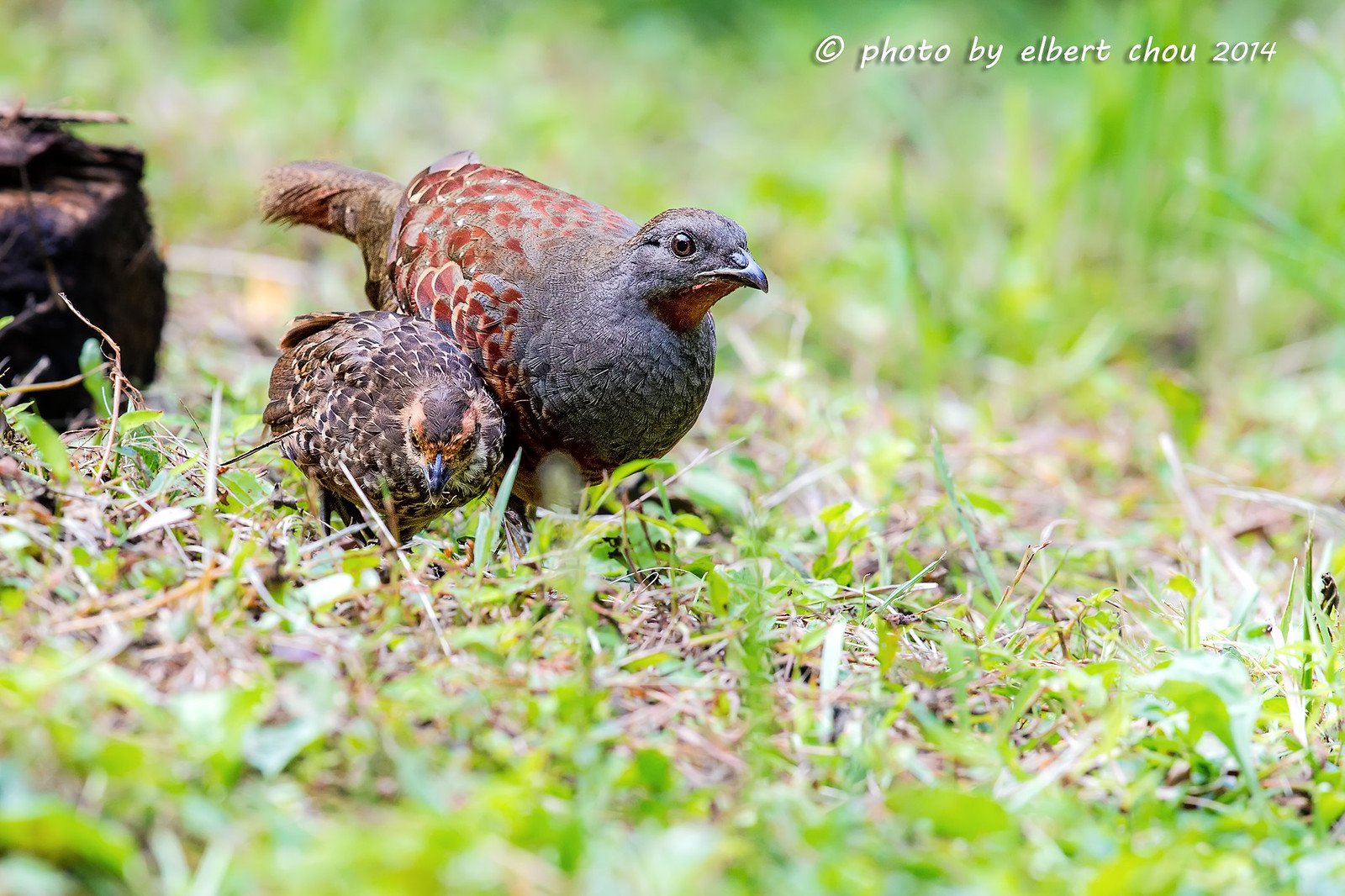This wide rectangular image showcases two birds on bright green grass, which is blurred at the top and bottom front. Twigs are interspersed among the grass. The larger bird, positioned near the center, faces diagonally towards the bottom left. It has a very dark grayish head and chest, transitioning to gray feathers with a bright reddish-brown pattern towards the back. Its tail is brown and flares out. In front of and slightly to the left of the larger bird is a smaller bird with uniformly brown feathers and a light brown face. Both birds seem to be wandering on the grass, surrounded by small blades, leaves, and twigs. Larger foliage is visible in the distance. The image is taken from a grass-level perspective. The top right corner shows a photo credit: "Copyright Photo by Albert Chao, 2014."